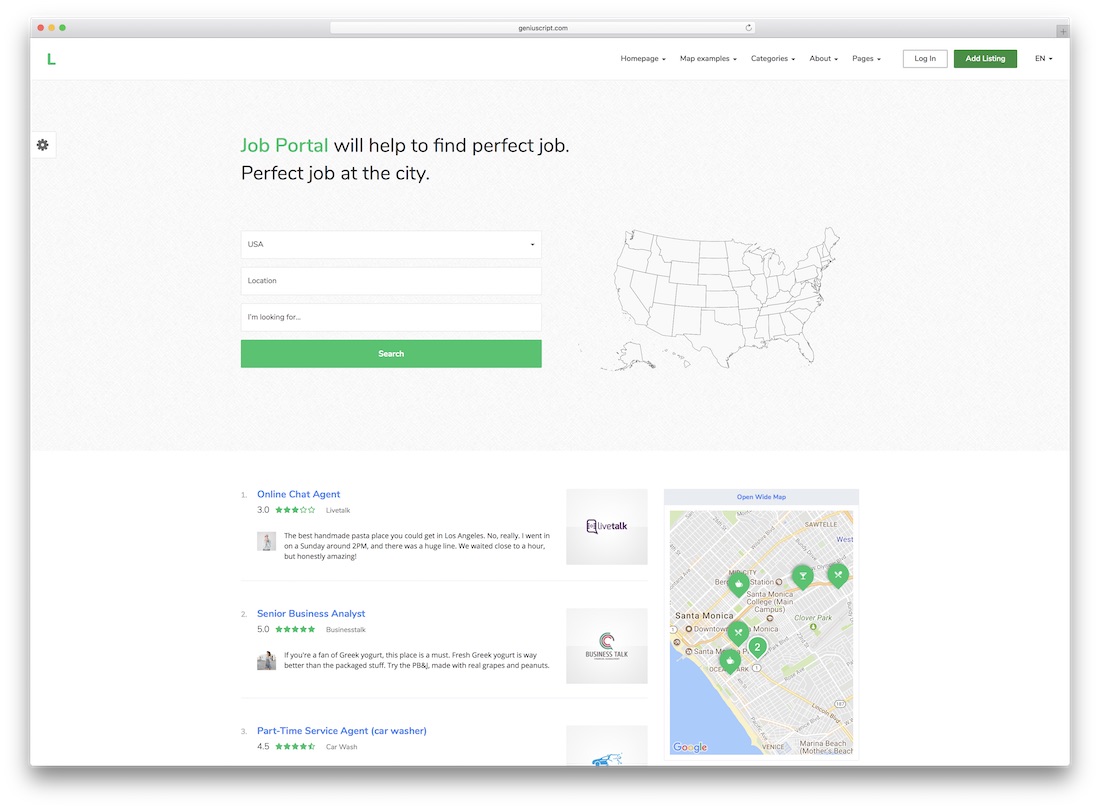A screenshot of a job portal web page is displayed. At the top, there's a white border with a green "L" logo in the upper left corner. On the right side of this border is a navigation menu featuring items labeled "Homepage," "Categories," and "About," along with two indistinguishable options. Next to the menu is a white "Login" button and a green button with unreadable text. Below, a headline reads, "Job portal will help to find the perfect job, perfect job at the city."

Continuing, there are three text input fields accompanied by a large green "Search" button. On the right side, there's a map of the United States. Below this section, a white area contains three distinct items written in blue, each accompanied by a star rating and explanatory text beneath them. Following this, the page features three gray text boxes, and finally, a box showcasing a screenshot of a map.

This detailed description captures the various elements and layout of the job portal webpage, providing a clear vision of its structure and content.